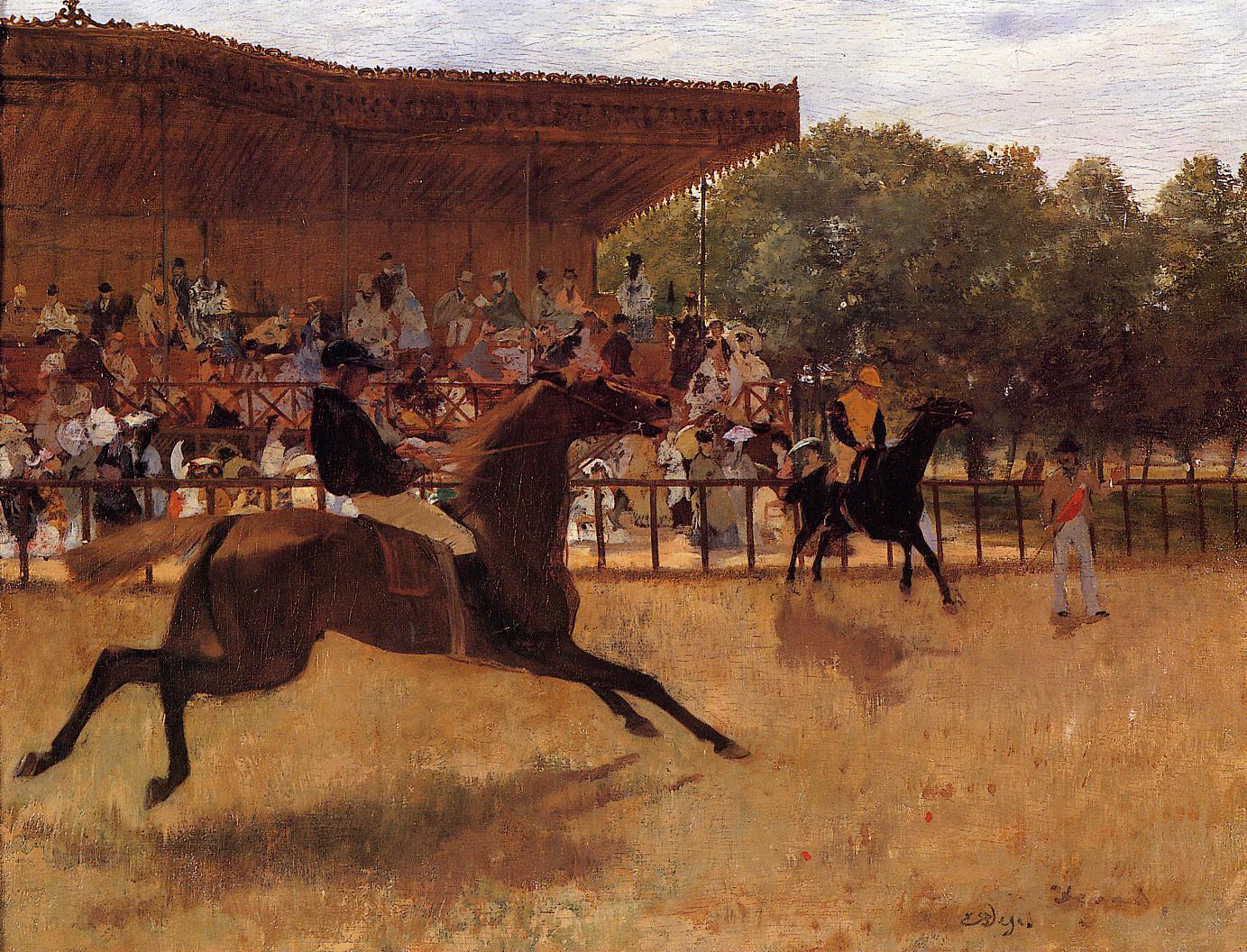This hand-painted artwork showcases a vivid and textured scene depicted on a large square canvas. The upper portion of the painting is dominated by a textured blend of blue, white, and hints of red, representing a sky interspersed with some clouds and possibly trees. Below the sky, a structure resembling a large, open-sided wooden pavilion is filled with numerous spectators who are either standing or seated. The pavilion forms the backdrop, with a fence sectioning off the foreground from the background.

In the foreground, the ground is depicted with a blend of dark brown and light brown patches, representing dirt mixed with brown grass. The most dynamic element in the painting is a scene with two horses. On the middle left side, a brown horse is captured mid-leap, with its rider dressed in a black helmet, black shirt, and beige pants tucked into black boots, leaning back in his seat. To the right, a black horse appears in motion, accompanied by a rider donning a yellow vest, black shirt, beige pants, and boots, along with a yellow cap. In front of the black horse stands a man wearing white pants, a black hat, and a brown top, holding what looks like an orange umbrella in one hand, waving the other.

The scene is set outdoors in the middle of the day, evident from the presence of natural light and clarity. The overall color palette includes shades of blue, white, green, brown, black, yellow, orange, red, and tan, providing a rich and lifelike depiction. The composition centers around the interaction between the horses, their riders, and the spectators, capturing a moment of vibrant activity and anticipation.